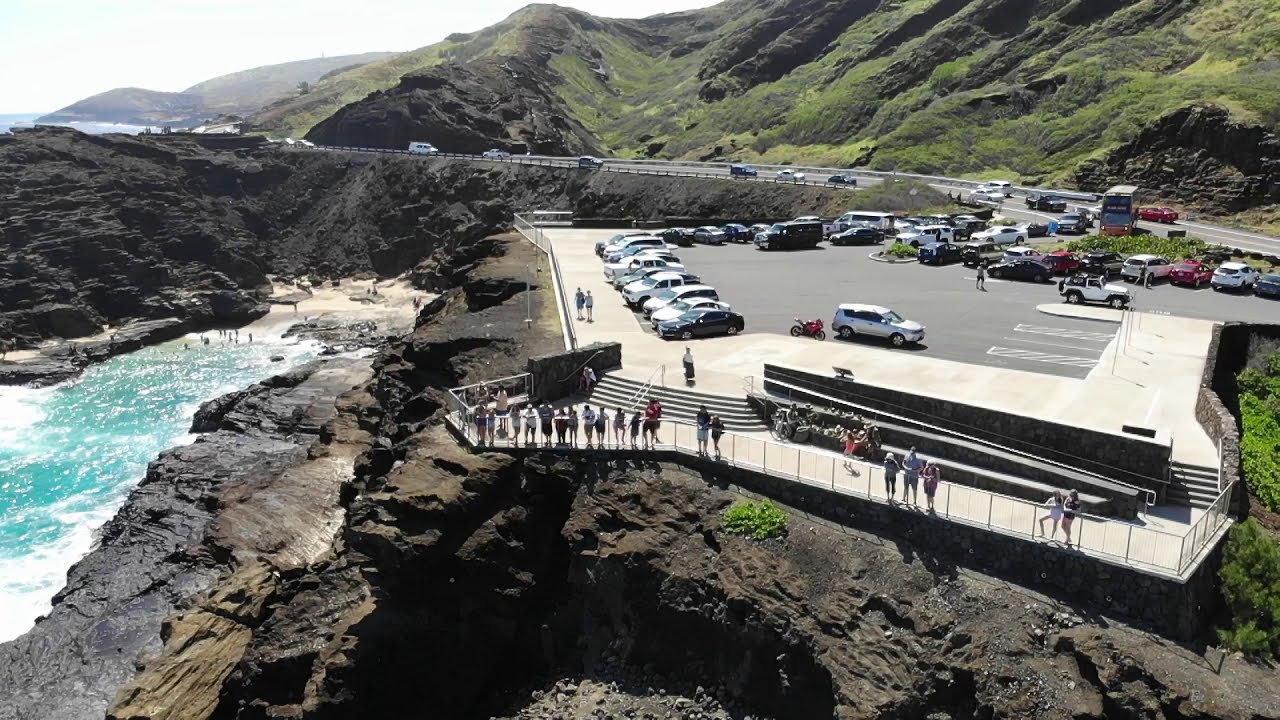This image captures a sharp, vivid scene of a scenic overlook nestled along a highway on a cliffside. In the foreground, a sizable parking lot, slightly off-centered to the right, hosts an array of vehicles including silver and white SUVs, a Jeep, and a large truck. Adjacent to the parking lot, a cement staircase and walkway lead to the cliff's edge, where a multitude of people lean against a fence, gazing downwards. The hilltops in the background are lush and green, with the road meandering through them, adding to the backdrop's splendor. Below the overlook, the dark black rock cliff descends steeply to meet the bright turquoise water of a lake or ocean, with a small beach cove where additional people can be seen wading in the water. The contrasting colors of green hills, brown rock formations, and vibrant blue water enhance the picturesque quality of this scenic site.